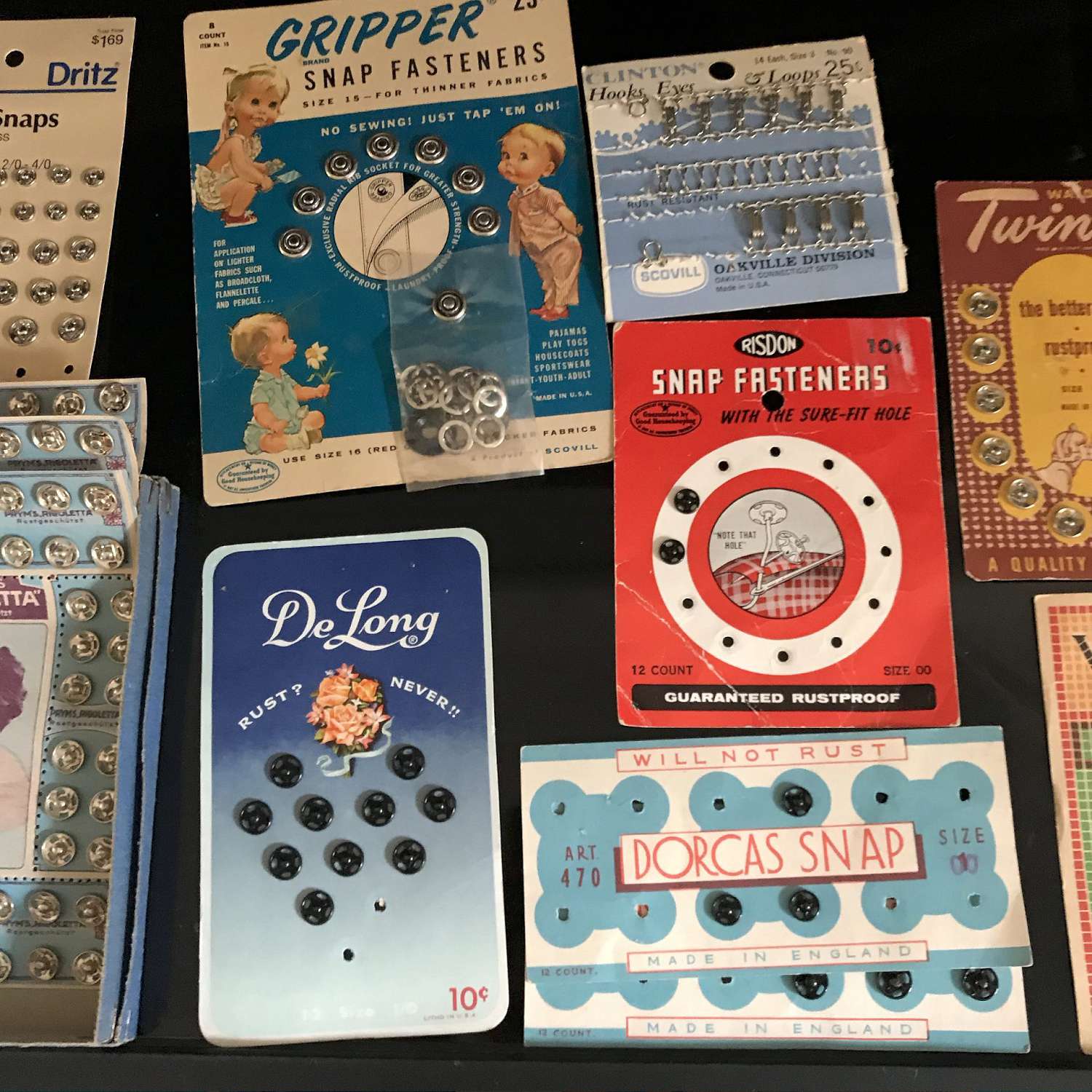This image showcases an assorted collection of vintage and retro snap fasteners and hooks, all preserved in their original packaging. The background appears to be a dark, bluish-black fabric, providing a stark contrast to the varied colors and designs of the packages.

At the top left, there are several "Gripper Snap Fasteners" displaying the message "No sewing, just tap them on," and featuring images of infants, suggesting they may have been marketed for baby clothing. The packaging is notable for the phrase "guaranteed rust-proof." 

In the bottom left, the "DeLong" snap fasteners are arranged in a pyramid formation, with the text "Rust? Never!!" and a price of 10 cents. Despite the passage of time, the package only has a few missing snaps.

Adjacent on the right is a red package of snap fasteners, marked by the slogan "Sure fit hole, 10 cents," also assuring that they are rust-proof. Below this, we see the "Dorcas Snap Fasteners," which are on blue-and-white packaging, declaring "Will not rust" and identified as "Art 470, Size 0." These fasteners are made in England, a detail highlighted prominently.

Also included in this vintage collection are "Clean Hunk Eye Loops," sold for 25 cents and distinguished by their silver color.

This detailed image offers a nostalgic glimpse into past everyday items, emphasizing their durability with repeated promises of being rust-proof.